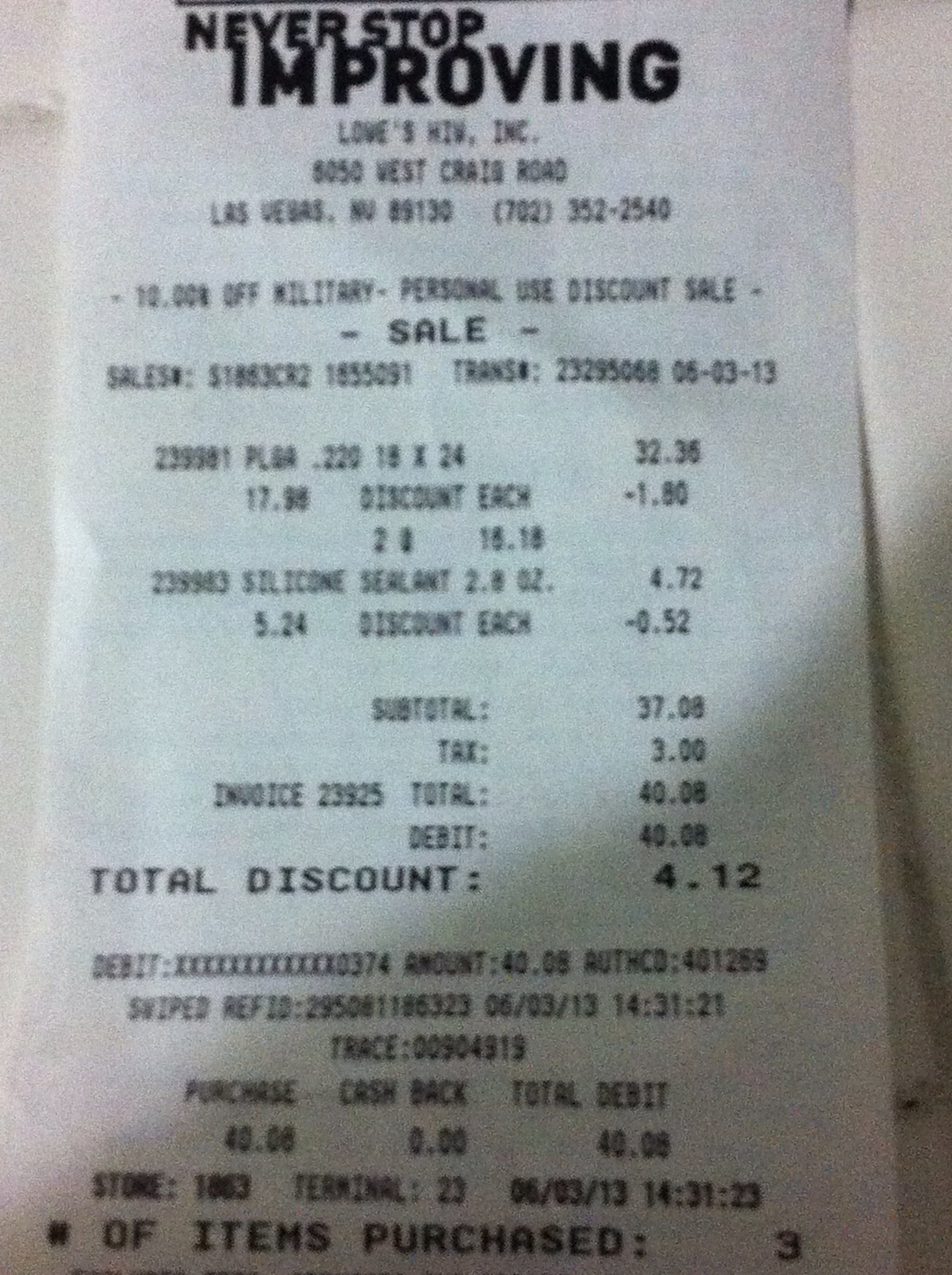This detailed description outlines the key elements visible in an image of a receipt:
 
At the top of the receipt, the phrase "Never Stop Improving" is prominently displayed in bold letters, serving as an optimistic slogan. Below the slogan, the store name "Loves" is visible, followed by "HIW Incorporated." The receipt also lists the store's address, "8050 West Craig Road, Las Vegas, Nevada," and provides a contact number, "702-352-2540."
 
Notably, there is a mention of a "10% off military personnel discount" offer, reflecting the store's support for military service members. The word "Sale" is prominently featured below the discount information, indicating that the purchases were part of a promotional event.

Further down the receipt, the purchase details reveal that two items were bought: one priced at $17.99 and the other at $5.24.